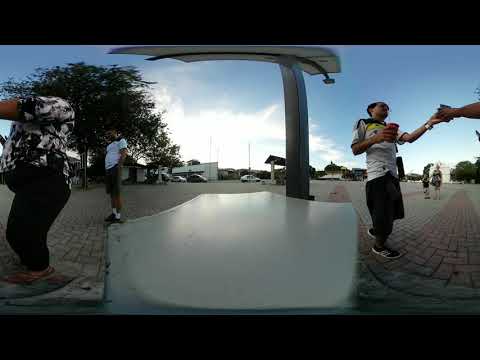This photograph, captured in a fisheye view, depicts an outdoor setting on a large concrete or brick plaza, bordered by a thick black frame on the top and bottom. The scene unfolds on a brick sidewalk made up of grey and red rectangular bricks. The sky above is predominantly blue with some white clouds scattered across, suggesting a daytime setting.

At the forefront, a silver pole stands at the center amidst a group of people who are interacting on the bustling street. Towards the left, a person clad in black leggings, pink tennis shoes, and a black and white patterned shirt is partially visible, with only the lower part of their body seen. Behind this individual, another person is dressed in a white short-sleeve shirt, dark shorts, and dark shoes paired with white socks.

On the right side, a person in a white, yellow, and black short-sleeve shirt, black pants, and black tennis shoes is depicted holding a drink in one hand while extending his other hand towards another person who is out of frame. This same figure is also noted to be interacting with another individual who is wearing a white shirt with dark camouflage patterns and black pants, indicating some exchange taking place.

The overall scene is enriched by additional elements such as passing vehicles, nearby trees, buildings, and various people walking or standing around, lending a lively atmosphere to the concrete plaza. There is also a noticeable large white, smooth object with a shiny surface at the image's center, accompanied by a metal pole, hinting at a possibly robotic structure that the camera might be mounted on, adding an intriguing dimension to the image.